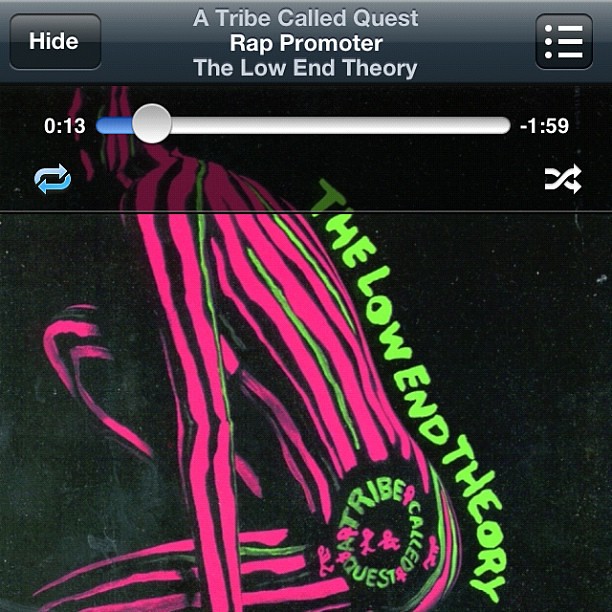This image depicts a music player app interface featuring an album cover as the background. The background showcases an abstract side view of a woman in body paint, predominantly black with striking pink and green stripes along various parts of her body. Her pose is distinct, with her right leg folded up towards her chest, and the words "A Tribe Called Quest" marked on her thigh area. Running along her back in green letters is the phrase "The Low End Theory." The upper half of the screen is dominated by the app interface. At the top, there's a gray border with a "hide" button on the left, followed by the text "A Tribe Called Quest - Rap Promoter - The Low-End Theory" centrally positioned. To the right of this gray bar is a menu icon. Below this header, a progress bar shows the length of the song, starting at 0:13, with a little blue section indicating the elapsed time, and ending at -1:59. The interface also includes replay and shuffle buttons enhancing its functionality.